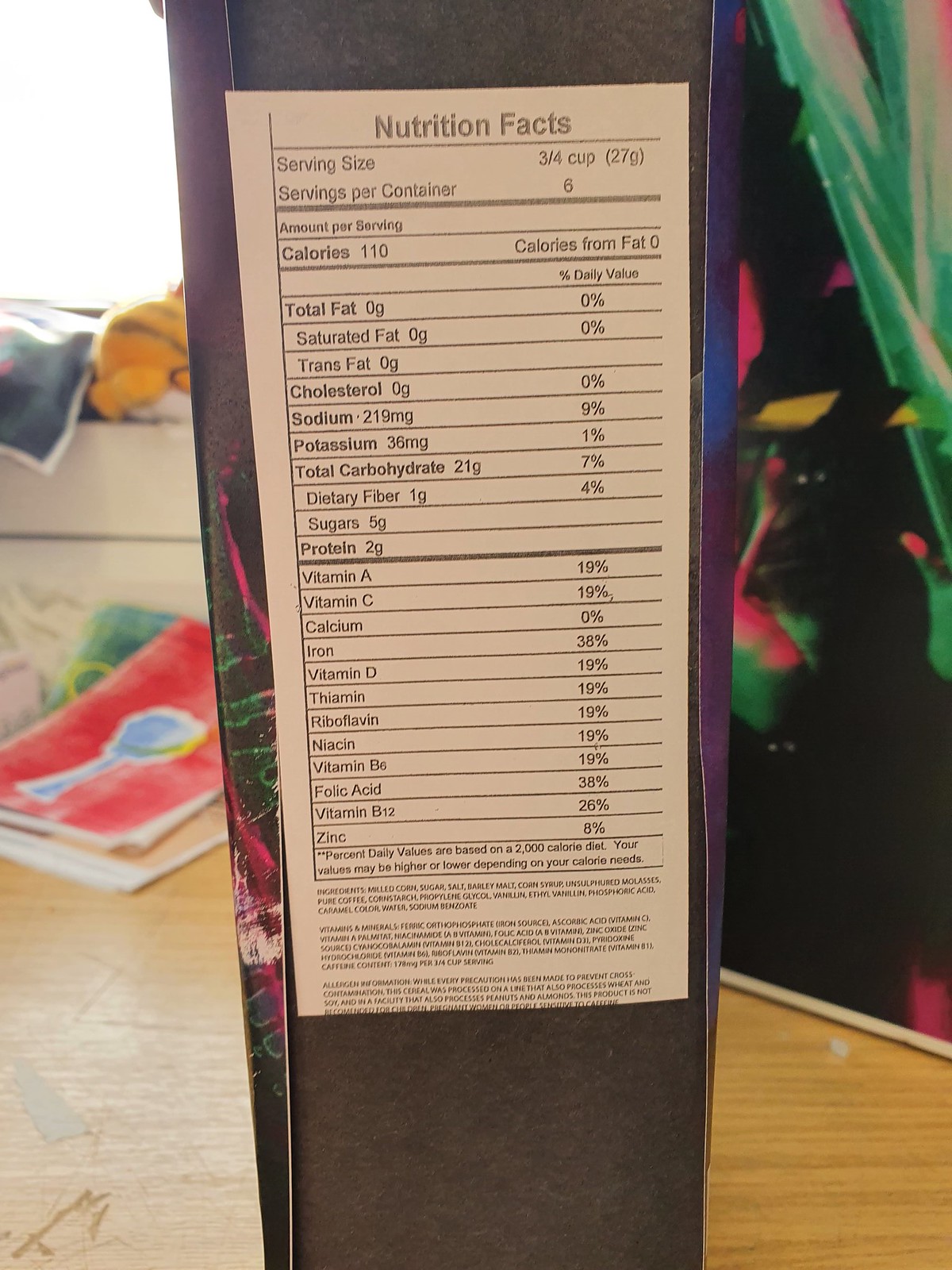This image depicts the side of a black, purple, and pink product box displaying a Nutrition Facts table. The box is placed on a wooden surface. The Nutrition Facts table is white with black text and reads: "Serving size: 3/4 cup (27 grams), Servings per container: 6." The nutritional information includes: "Calories: 110, Calories from fat: 0, Total fat: 0g, Saturated fat: 0g, Trans fat: 0g, Cholesterol: 0mg, Sodium: 219mg, Potassium: 36mg, Total carbohydrates: 21g, Dietary fiber: 1g, Sugars: 5g, Protein: 2g, along with amounts for Vitamin C, Calcium, Iron, and Vitamin D." In the background on the left side, a Garfield stuffed toy is visible, with some colorful drawings or paintings below it. On the right side, there is a costume with green, black, yellow, and pink colors. Brightly colored papers in red, blue, and peach are also seen behind the box.